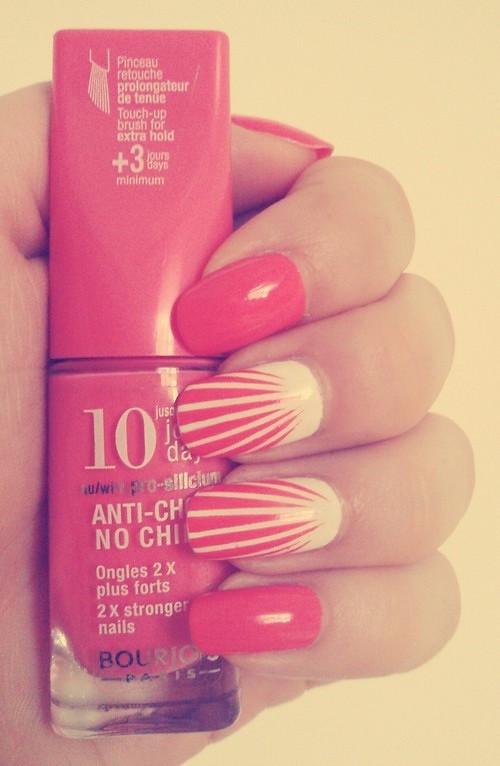In this detailed close-up image, a woman's hand, adorned with well-manicured nails, holds a bottle of nail polish. The background features a simple beige wall that contrasts with the vibrant colors in the foreground. The bottle itself is distinct, with a pink cap and a clear glass bottom, allowing a full view of the pink polish inside. The detailed text on the bottle includes the phrases "touch up brush for extra hold plus three days minimum," "10 pro-silicone," "anti-chip," "two times stronger nails," all in both English and French, such as "Pinceau Retouche Prolongateur de Tenue" and "3 Jours minimum D'Aise."

The hand's nails are painted in a striking manner—most are a solid pink, while the middle and ring fingers feature a creative design with white bases and pink stripes that resemble rays of light emanating from the nail bed. The polish on her nails is glossy, adding to the overall polished appearance of the image. The product branding includes "Maurice Paris," adding a touch of elegance and sophistication to the scene.